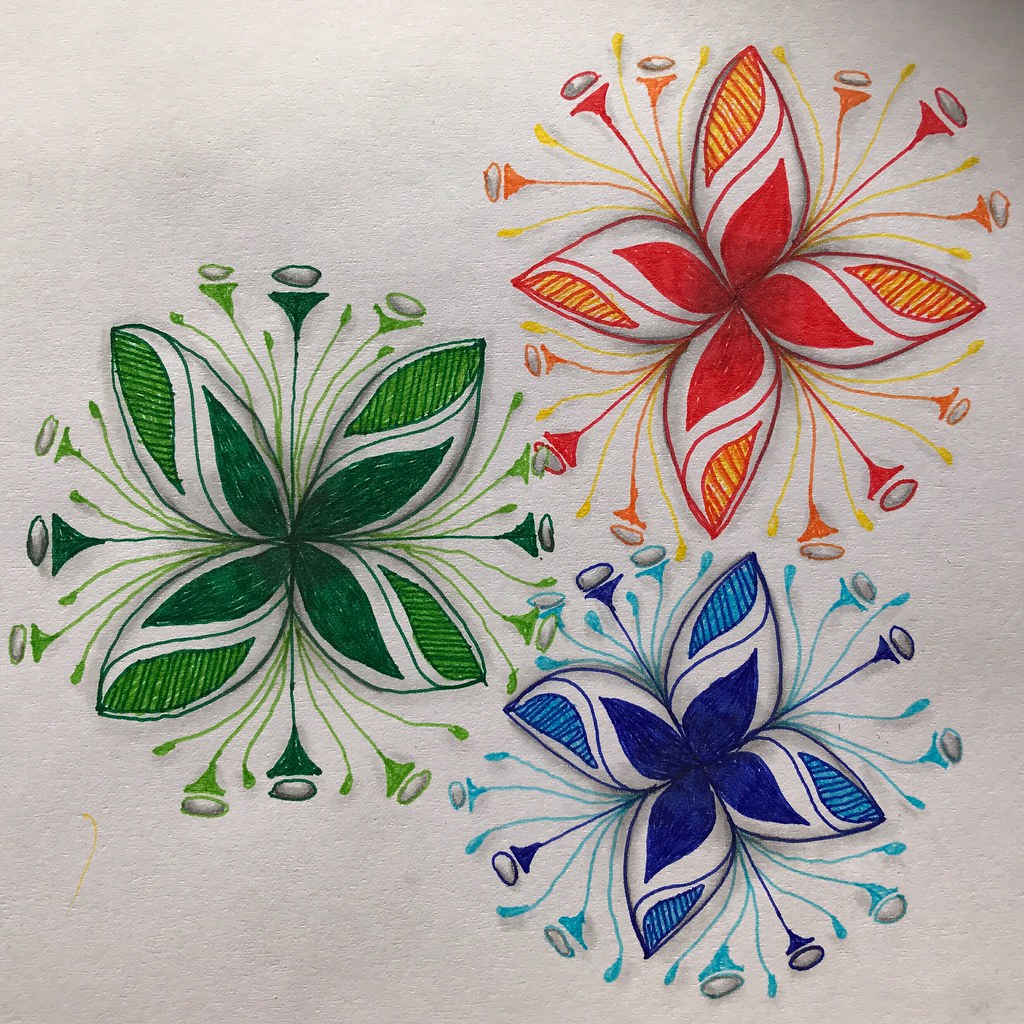The image showcases a detailed colored pencil drawing of three distinct yet similar flowers, presented on a white piece of paper. Each flower features four slightly pointed petals that are rounded in the center, with reproductive parts including filaments or anthers extending from the gaps between the petals. The flowers vary in color: one is predominantly green with a green and white swirl effect on its petals and small green and white spherical structures growing from the stems. Another flower is a combination of orange, red, and white with similar white swirls and red accents. The third, slightly smaller flower is blue with white swirls on the petals and blue stems with white spherical end points. All three flowers share the common theme of multicolored petals with intricate details, creating a cohesive yet vibrant floral composition.